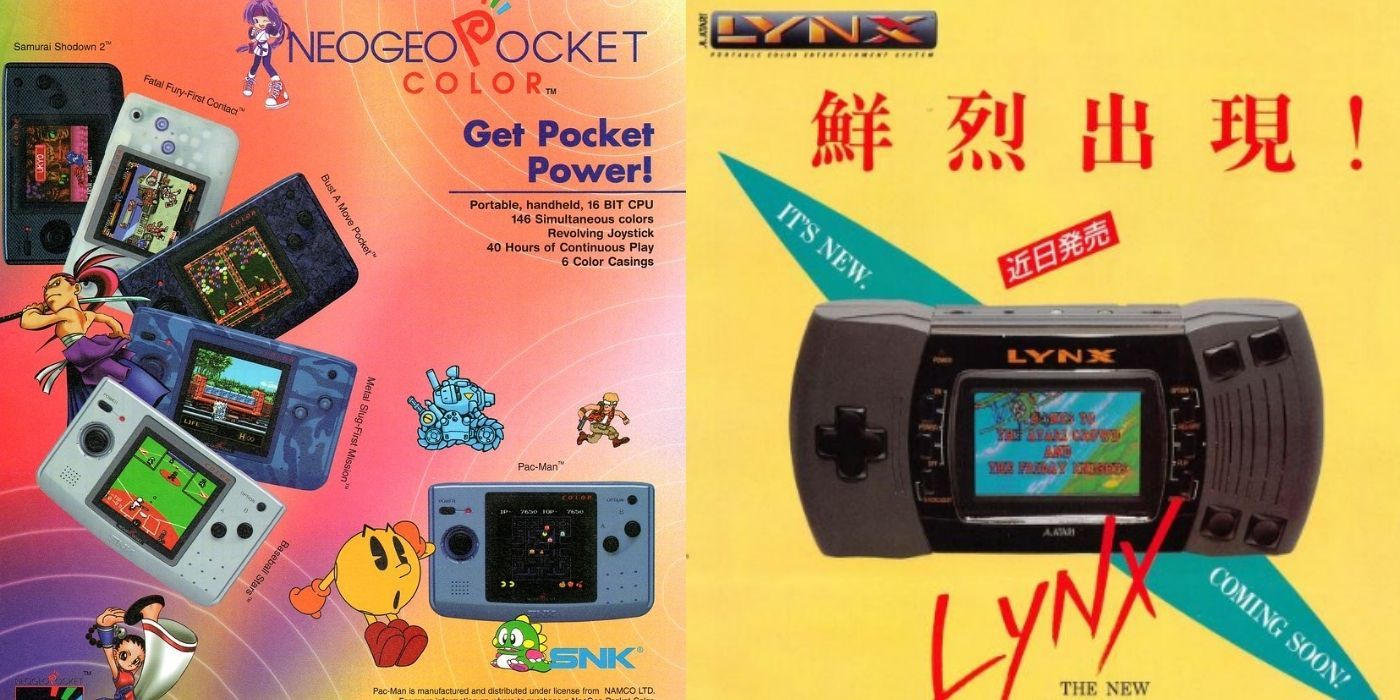This digital advertisement showcases two sections featuring handheld game consoles side by side. The left section, vibrant and busy, displays a colorful background dominated by pink, with accents of purple in the lower left and yellow in the lower right. At the top, bold text reads "Neo Geo Pocket Color" followed by the slogan "Get Pocket Power." Below this, smaller text details the console's features: "Portable Handheld, 16-bit CPU, 146 simultaneous colors, revolving joystick, 40 hours of continuous play, 6 color casings." The left section also includes staggered images of the console, surrounded by various cartoon figures.

The right section features a solid yellow background with four large red symbols at the top, indicating "Happy New Year" (新年祝生) in Chinese, followed by an exclamation mark. Below, the center showcases a digital screen displaying the game console "Lynx" (spelled L-Y-N-X) with its interface. On the left side of the controller, a black cross-shaped directional pad is visible, while two black buttons are positioned in the upper right and lower right corners. Diagonally across the bottom of this section, the text "Lynx" is prominently featured again, with the accompanying phrase "It's New Coming Soon" positioned against the yellow background.